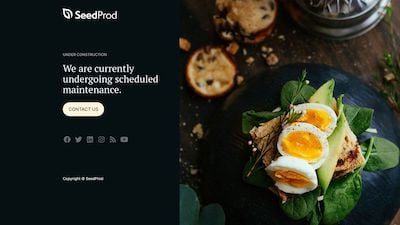The image features a webpage under the brand "Seed Prod" with a prominent "Under Construction" notice indicating scheduled maintenance. The left side of the page, set against a black background with white text, includes a "Contact Us" button in beige with black text, and a row of social media icons including Facebook, Twitter, Indeed, Instagram, and YouTube. Below this section, there is a copyright notice in white text. The right side of the page showcases a vibrant image of a food item, likely a sandwich, featuring green leafy vegetables and sliced bread both in the middle and on top. The sandwich also appears to contain elements resembling an egg, with white and yellow components. The food is displayed on a wooden table strewn with assorted ingredients, suggesting a kitchen setting or a product focused on food. The wooden table is brown, complementing the colorful and appetizing food items which dominate the right portion of the webpage.